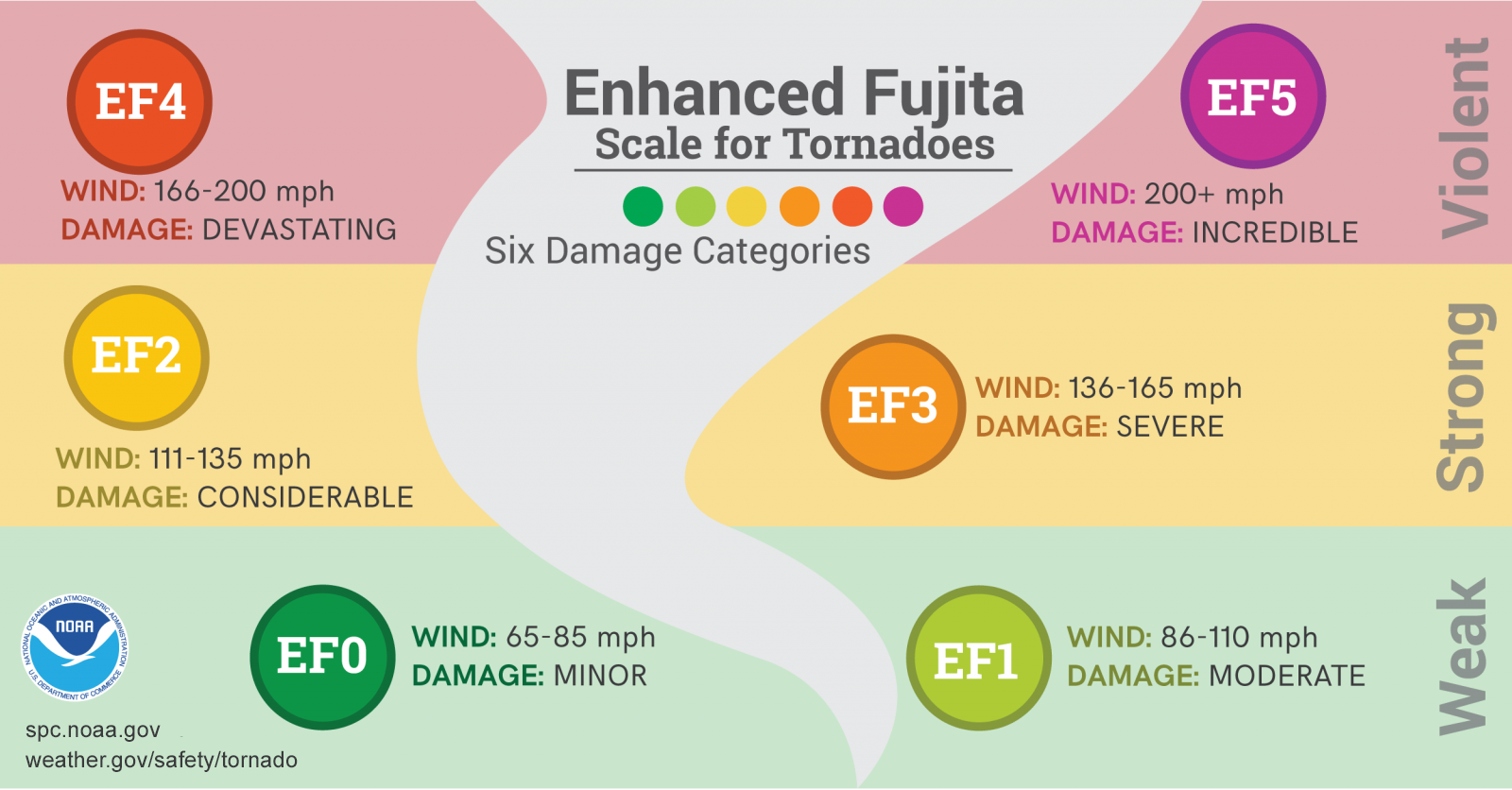This image is an infographic titled "Enhanced Fujita Scale for Tornadoes" that categorizes tornado damage into six distinct levels based on wind speed and severity. A stylized tornado graphic is centrally featured, with the categories represented by colored circles and arranged in a clear, tiered structure.

Starting at the bottom, EF0 is marked in dark green for weak tornadoes with wind speeds of 65-85 miles per hour, causing minor damage. Adjacent to it is EF1 in light green, denoting weak tornadoes with wind speeds of 86-110 miles per hour, leading to moderate damage.

Moving up, the middle tier features EF2 in yellow, representing strong tornadoes with wind speeds of 111-135 miles per hour, resulting in considerable damage. Next to it, EF3 is illustrated in orange, indicating strong tornadoes with wind speeds of 136-165 miles per hour that cause severe damage.

At the top, EF4 is designated in red for violent tornadoes with wind speeds of 166-200 miles per hour, causing devastating damage. EF5, portrayed in purple, denotes the most severe tornadoes with wind speeds exceeding 200 miles per hour, resulting in incredible damage.

The backdrop of the infographic is color-coded to emphasize the severity levels: green shades for weak categories, orange for strong, and purple for violent. On the left side, the NOAA seal is visible, along with a link to their website for further information on tornado safety. This poster serves as a comprehensive visual guide to understanding the Enhanced Fujita Scale and the corresponding damage potential of tornadoes.